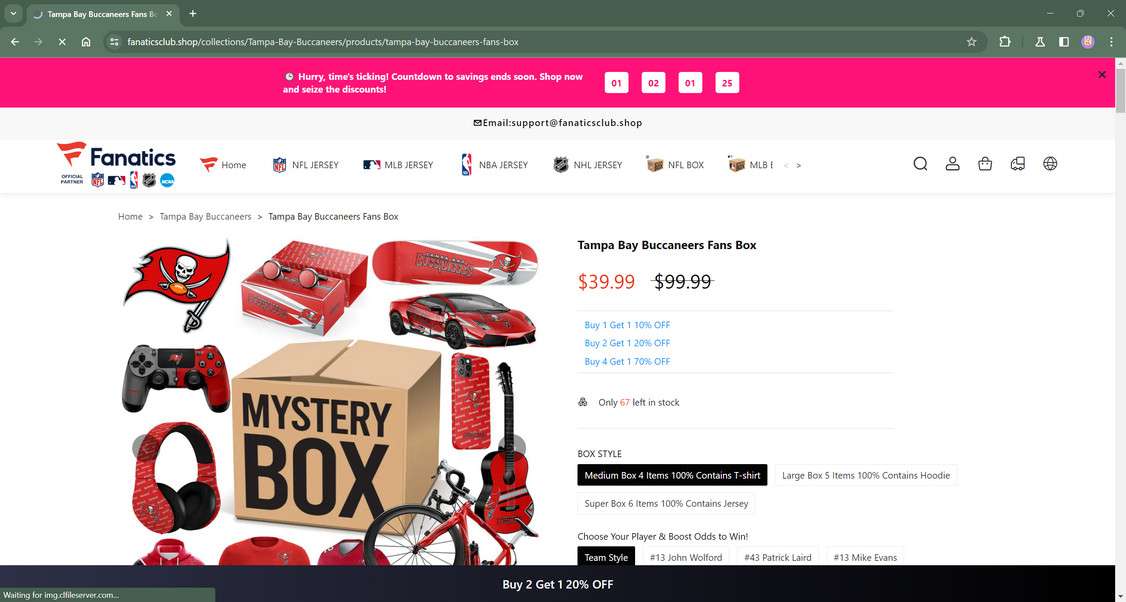The image features a multi-faceted digital flyer designed with a light blue background. At the top left corner, there is a small black box with a down arrow and very tiny white text inside, accompanied by a search box, an "X", more small icons, and another search box, followed by more icons with a hint of pink at the end.

In the center is a prominent bright pink box with a circular text element inside that reads "Hurry! Time’s a-ticking! Countdown to savings ends soon." Below this, there is a "Shop now and save" prompt followed by four small white boxes each containing numbers. A black "X" is placed at the end of this section.

Beneath this, a blue box contains a small square and the email support information: "support@fanaticsclub.shop." Following this is a white section labeled "Fanatics" with a small red flag icon and several navigation icons beneath it. Categories listed include "Home," "NFL Jersey," "MLB Jersey," "NBA Jersey," and "NHL Jersey," alongside respective search boxes and icons.

Further down, a white background features a collection of Tampa Bay Buccaneers merchandise in red, including a flag, cufflinks or earrings, a car, a guitar, a bicycle, and headphones. Notably, a "Fans Box" is priced at $39.99, with a stock count of only 67 left. Towards the bottom, another black box contains text and is followed by a longer black box offering a "Buy two, get one 20% off" deal.